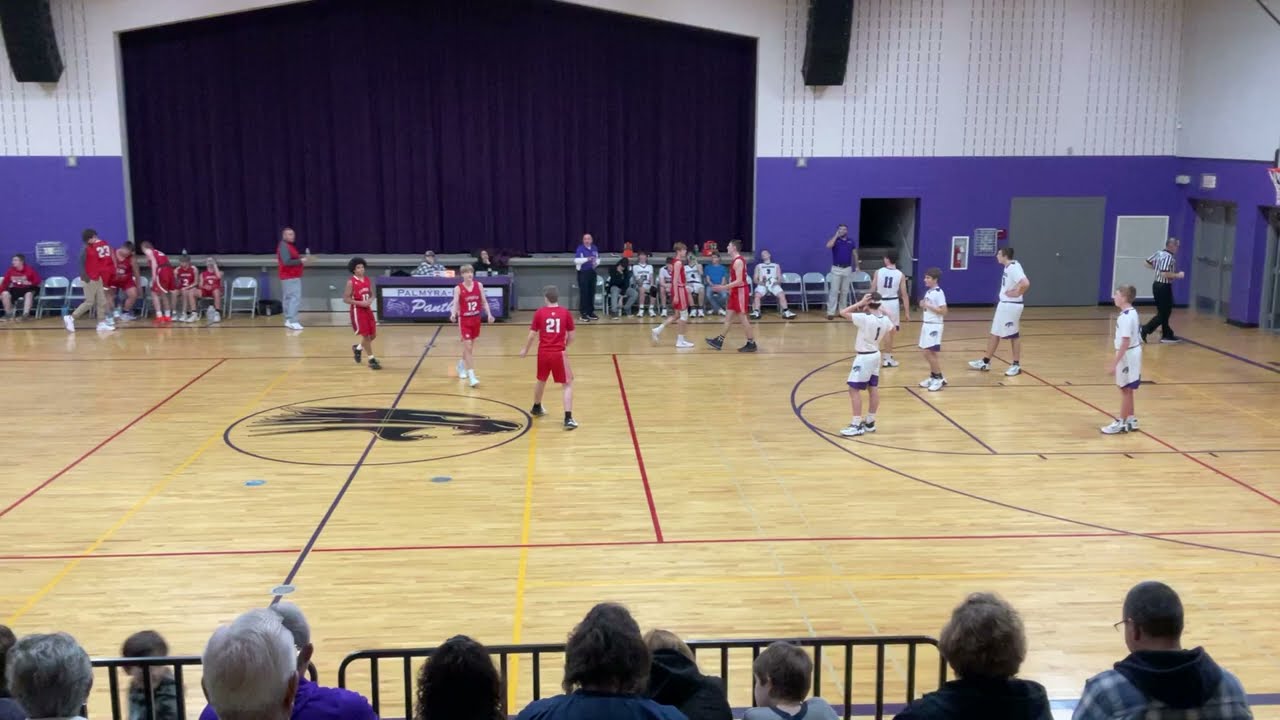This image captures the vibrant scene of a high school basketball game taking place in a spacious gymnasium distinguished by its distinctive purple and white decor, which suggests that the team in white with purple trim is the home team. The basketball court features multiple colored lines, including purple for basketball and red and yellow for volleyball, along with a central logo depicting a panther. 

The game seems to be in a brief timeout as evidenced by the players from the team in red and the team in white and purple getting into position—the players in white are in the key area under the basket while the red-uniformed players are scattered around midcourt with some walking onto the court. 

Spectators' heads line the bottom of the image, indicating they are seated along the sidelines, with a guardrail separating them from the court. On the opposite side of the court, benches along with coaches and reserve players can be seen. Behind them, a large stage with a dark purple curtain adds depth to the background, alongside a score table and referees preparing to resume the game. The walls of the gym are primarily white with a blue section at the bottom, completing the dynamic and bustling atmosphere of the scene.